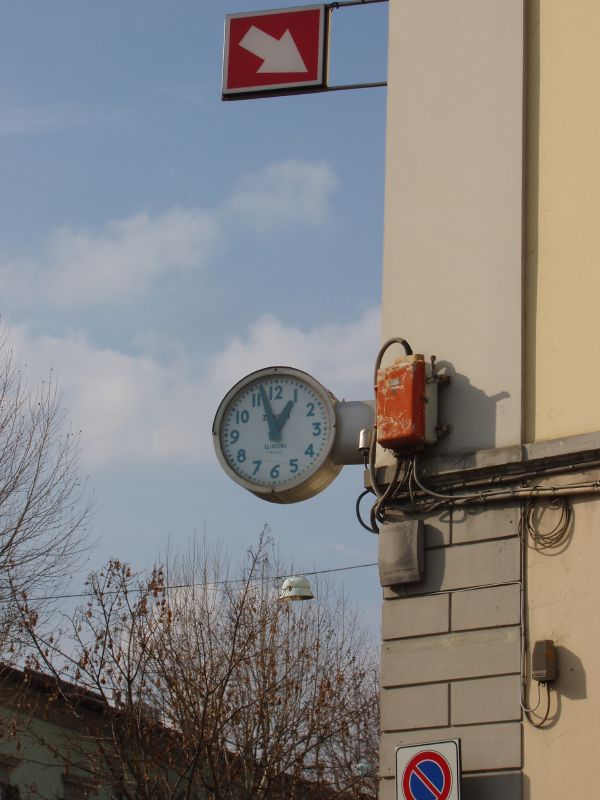The image is a detailed color photograph of the corner of a building taken from a low angle. The lower part of the building corner shows a brick pattern, giving it a textured, stacked brick appearance while the upper part is smooth and plain white. Occupying a central position on this corner wall is a metal-housed clock, securely mounted by a small, round gray connector. The clock, featuring a white face with black numbers and rounded black hands, reads approximately 12:57. Affixed further up the corner wall, several feet above the clock, is a red square sign with a bold white arrow pointing downward and to the right. Additionally, there are numerous electrical cords and conduits running along the wall, potentially leading to an electric box that powers the clock and possibly other devices. In the bottom corner of the image, there's a "Do Not" sign with a blue circle and a red slash, although what is prohibited is unclear. To the left, the image captures the tops of small trees silhouetted against a blue sky dotted with clouds.